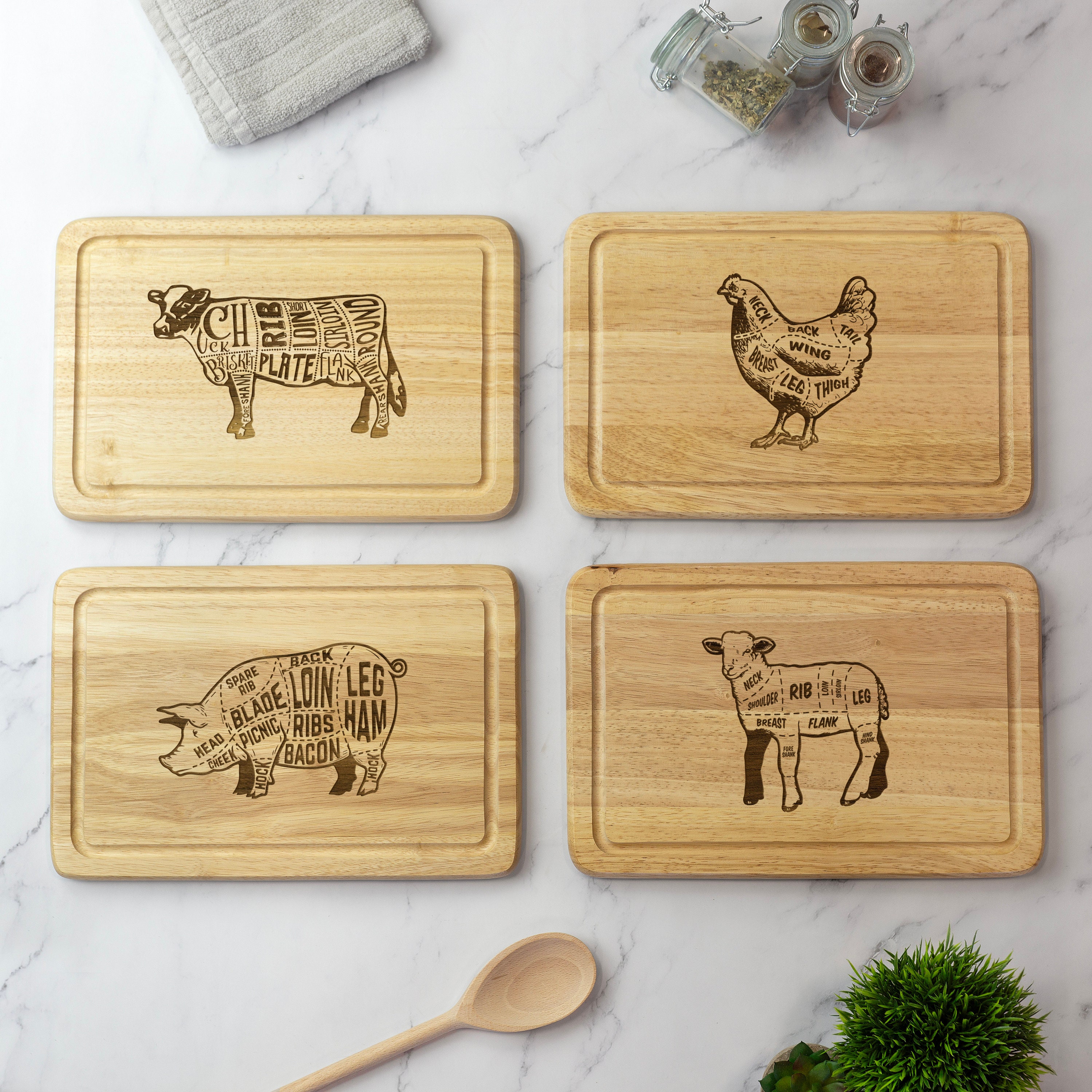The image depicts an overhead view of a marble countertop or tabletop with gray veining. Central to the composition are four rectangular wooden cutting boards, each featuring engraved graphics of a different farm animal segmented into its respective cuts of meat. The top left cutting board displays a cow with labels such as rib, loin, plate, and sirloin. To the right, the top right board showcases a chicken, similarly sectioned and labeled. The bottom left cutting board illustrates a pig with parts labeled as blade, loin, leg, and ham, while the bottom right cutting board features a sheep or lamb, marked with sections like rib and leg. 

Surrounding the cutting boards, several items are positioned to enhance the scene: at the top right corner, three glass containers filled with various spices, one of which is tipped over, revealing green spices. The top left corner holds a folded gray dish towel. At the bottom of the image, a wooden spoon and a green house plant add a touch of natural texture and color contrast to the setup. The cutting boards themselves are made of blonde wood with darker brown grains and have a groove running around their edges.